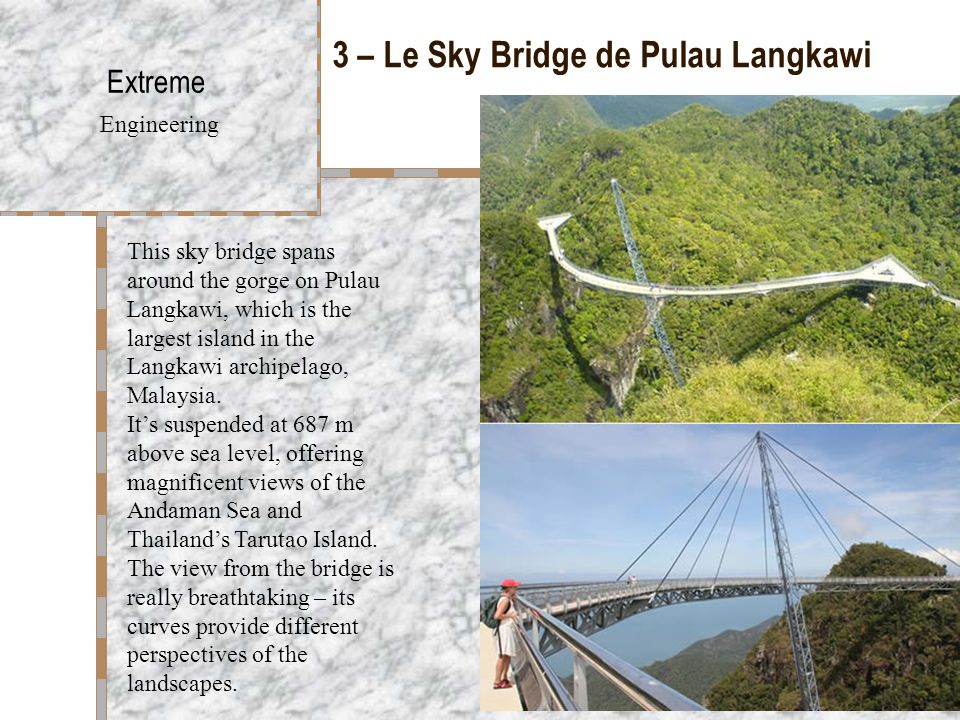This image displays a detailed illustration of the sky bridge on Pulau Langkawi, the largest island in the Langkawi Archipelago, Malaysia, known for its extreme engineering. The left-hand side features text on a black and white marble background, prominently titled "Extreme Engineering." Below, it describes the sky bridge as a remarkable feat spanning a gorge, suspended 687 meters above sea level. The bridge offers breathtaking views of the Andaman Sea and Thailand's Tarutao Island, with its curves providing varied perspectives of the lush landscape.

The right side of the image showcases two photographs of the sky bridge. The top photograph captures a panoramic view of the bridge set against a backdrop of verdant mountains and dense jungle, illustrating its white structure extending between two hilltops. The bottom photograph provides a close-up of the bridge, highlighting its architectural details and featuring a woman in a white dress and red hat gazing at the surrounding hills. The overall presentation, with its text and imagery, conveys the bridge’s engineering marvel and the stunning vistas it offers.